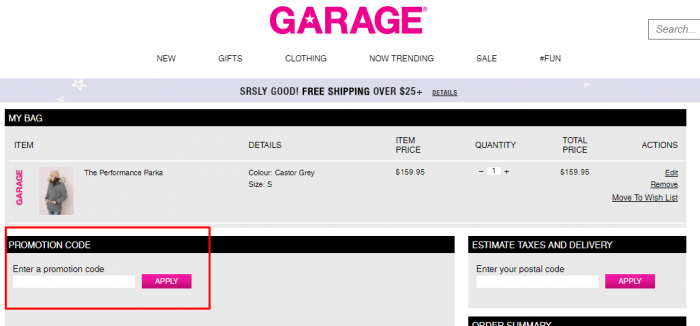The image depicts a webpage featuring an online store. At the top of the page, there's a navigation bar with categories such as "Garage," "New," "Gifts," "Clothing," "Now Trending," and "Sale." Additionally, icons and links for "Phone" support, a search function (top right), and an offer for "Free shipping over $25 plus details" are visible. On the top left, there is a link to "My Bag," which shows an item currently in the shopping cart: the "Performance Packer Apollo, Size: Small." The item is priced at $159.95, with a quantity of one in the cart. There's a field to enter a promotion code, which is highlighted in red, and options to estimate taxes and delivery costs by entering a postal code and applying the information. An order summary section is also present. The webpage's color scheme features shades of pink, red, white, grey, and black.